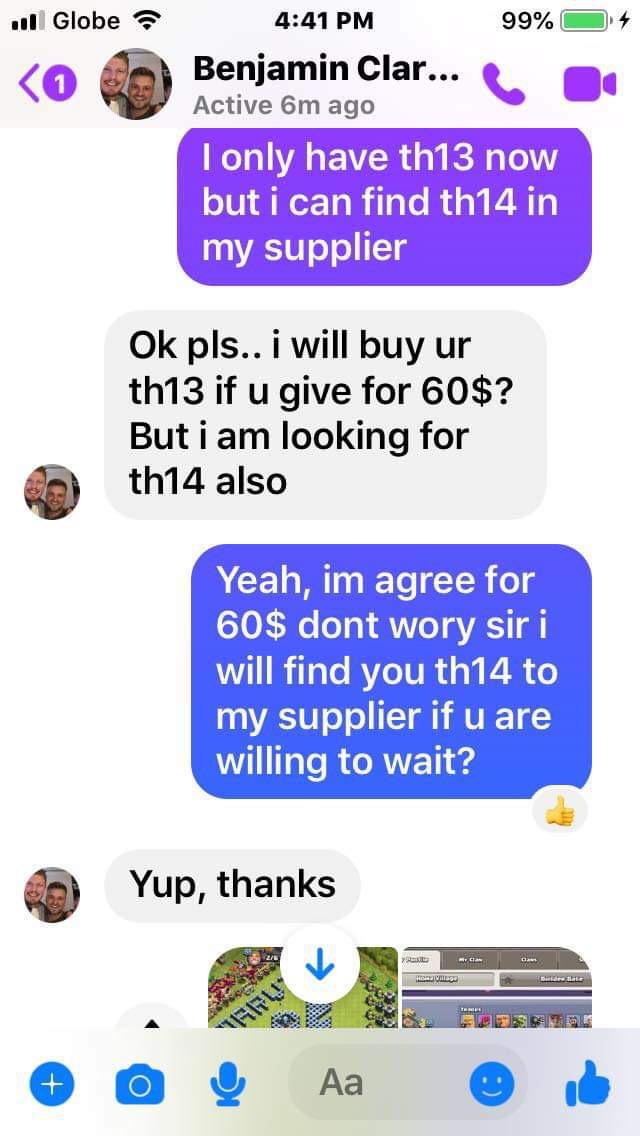This screenshot captures a text message exchange on a smartphone at 4:41 p.m. with the device connected to Wi-Fi and showing a 99% battery that is charging. The conversation involves the phone's owner and a contact named Benjamin Clark, with his last name cut off to "Clark...," indicating he was active six minutes ago. Benjamin's profile picture features two men with facial hair, one wearing a white shirt. The messages reveal a negotiation about procuring items labeled as "th13" and "th14." The owner states, "I only have th-13 now but I can find th-14 with my supplier," on a purple background. Benjamin responds with, "Okay PLS, I will buy your th-13 for $60 but I am looking for th-14 also," on a gray background. The owner then replies in blue text, "Yeah, I'm agree for $60. Don't worry, sir, I will find you th-14 with my supplier if you are willing to wait," followed by a thumbs-up from Benjamin and his reply, "Yep thanks." The exchange concludes with a partially visible image sent by the owner, indicated by a down arrow within a white circle, suggesting more content below. The messages contain noticeable spelling and grammar errors.